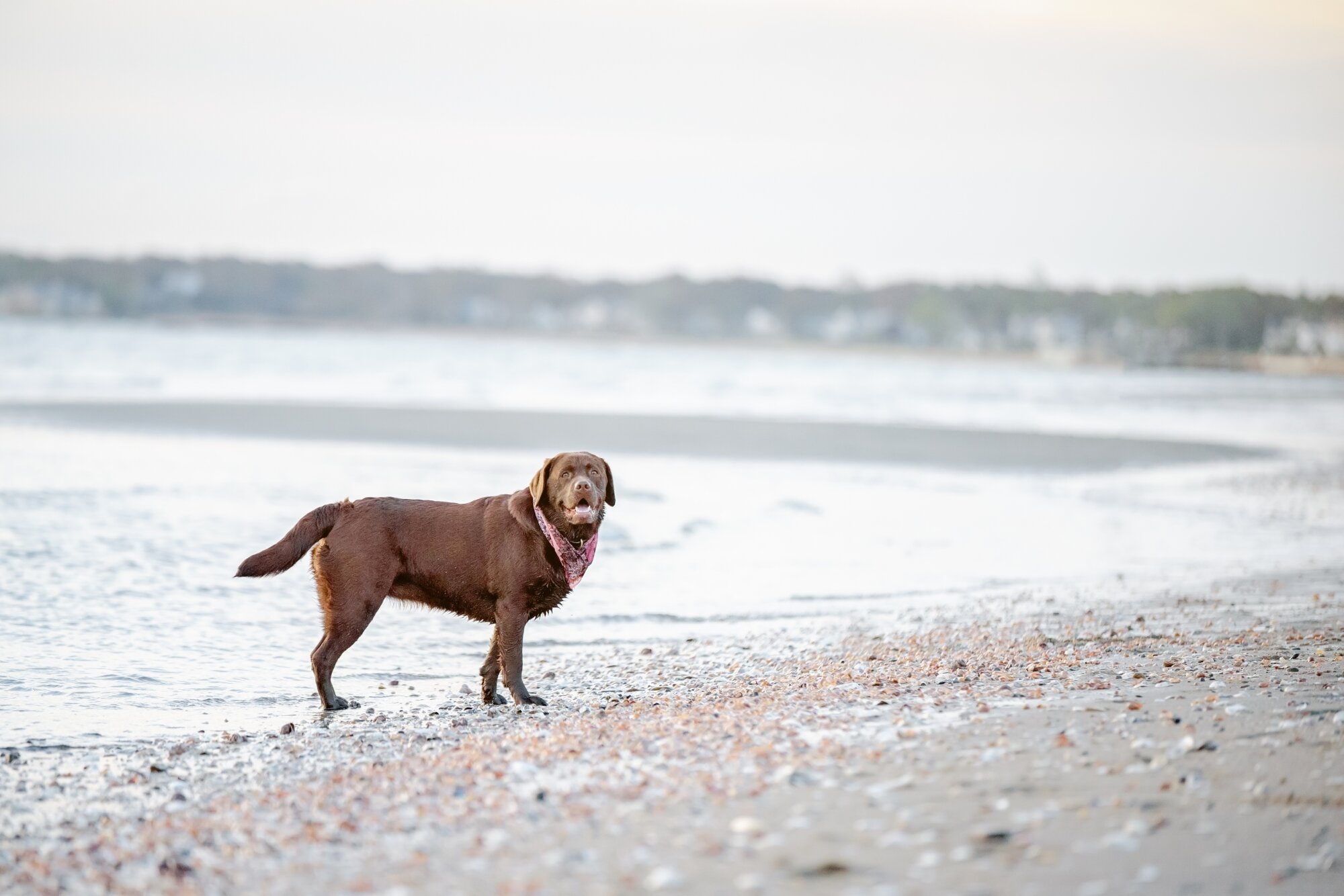In this photograph, there is a chocolate brown dog standing on a pebbly, slightly sandy beach near the water's edge. The dog, wearing a red bandana around its neck, has short hair, floppy ears, and a bulky frame with a thick tail held out behind. The dog appears to be smiling, with its mouth open and is looking directly at the camera, as if it was called by its owner while running. Its rear paws are partially in the shallow water, which glistens brightly under the daylight, while its front paws are on the sand mixed with seashells and rocks. The beach stretches out, showing signs of low tide with receded water. In the background, the green horizon is visible, along with a faint outline of residential homes. The overall scene is bright and almost devoid of other people, emphasizing the tranquil, open landscape with the dog being the focal point. The colors prominent in the image include various shades of brown, light red of the bandana, gray, light blue, green, and darker blue.